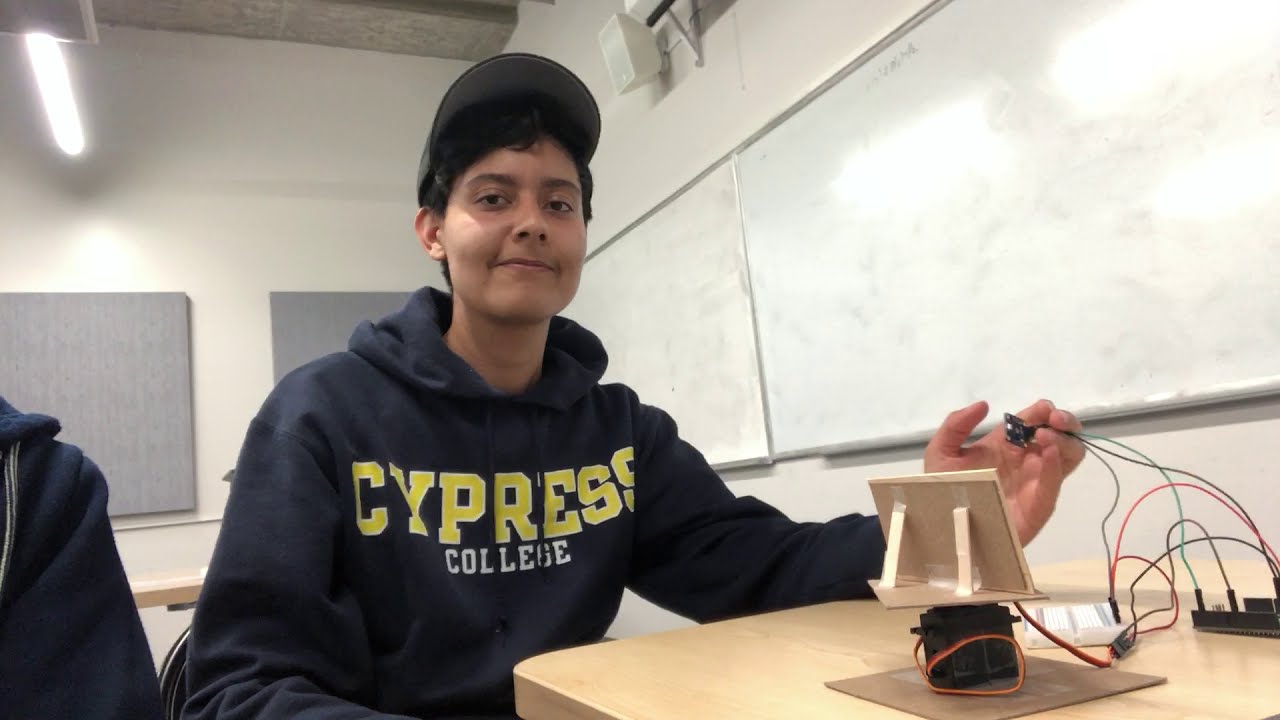The image shows a young man, likely around 19 or 20 years old, seated at a desk in a classroom environment, suggesting a science or electronics class. He has tan skin and short, dark-colored hair, and he is wearing a cap along with a navy blue sweatshirt that reads "Cypress College"—'Cypress' in yellow letters and 'College' in white. The young man is looking directly at the camera, with his left hand holding a project comprising several connected components, including red, green, and blue wires, attached to both white and black breadboards, possibly indicating an electronics experiment. Behind him are whiteboards and gray panels, and the classroom is bright, illuminated by a light in the top left corner of the image. The setting feels organized but focuses on the detailed project the student is handling at the wooden desk.